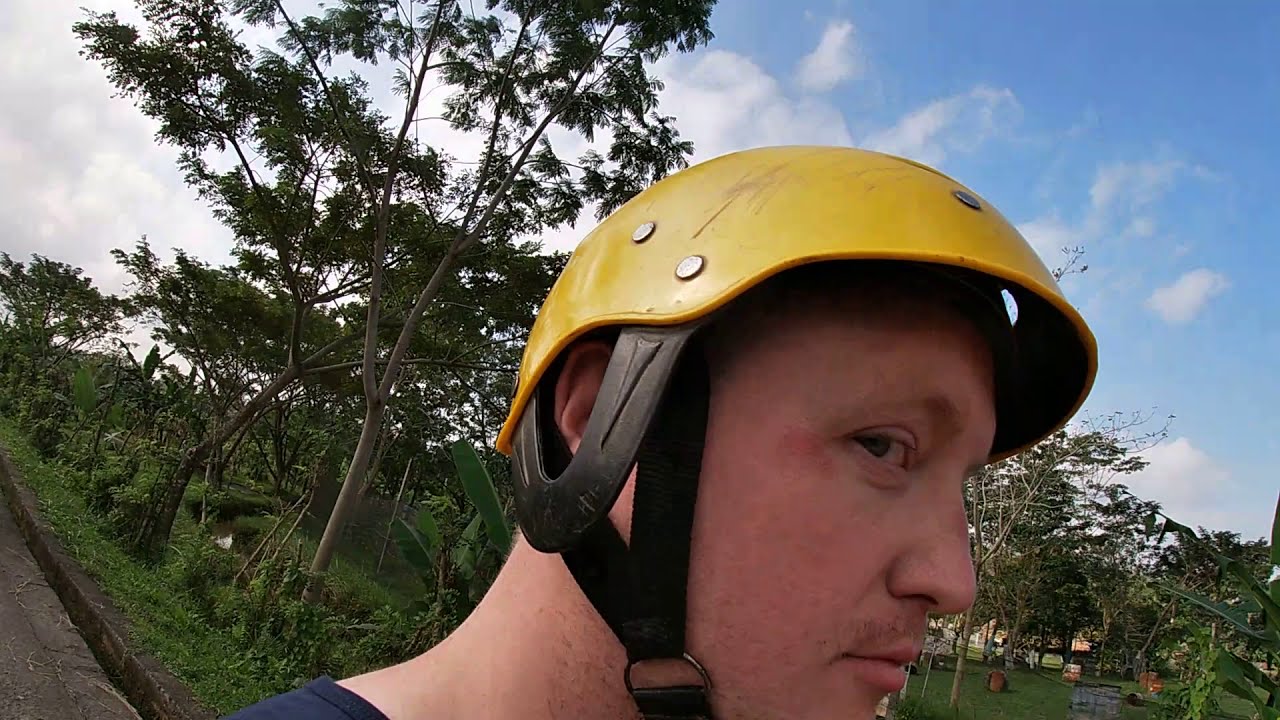This horizontally aligned rectangular image captures a close-up of the right side of a man's face, with his right eye turned towards the camera. He is wearing a sturdy-looking yellow bike helmet with black straps that connect at his chin, casting a protective vibe. The man has pale skin and a very thin brown mustache, and he appears to be on some sort of road or path, indicated by a visible textured curb. He is dressed in a navy blue shirt, with just the very top of his right shoulder in view. In the backdrop, on the left, tall trees with narrow trunks and green leaves can be seen alongside patches of green grass. The sky occupies the upper right-hand corner, clear blue with thicker patches of white clouds towards the left. On the far lower right corner, the landscape extends into more greenery and trees.